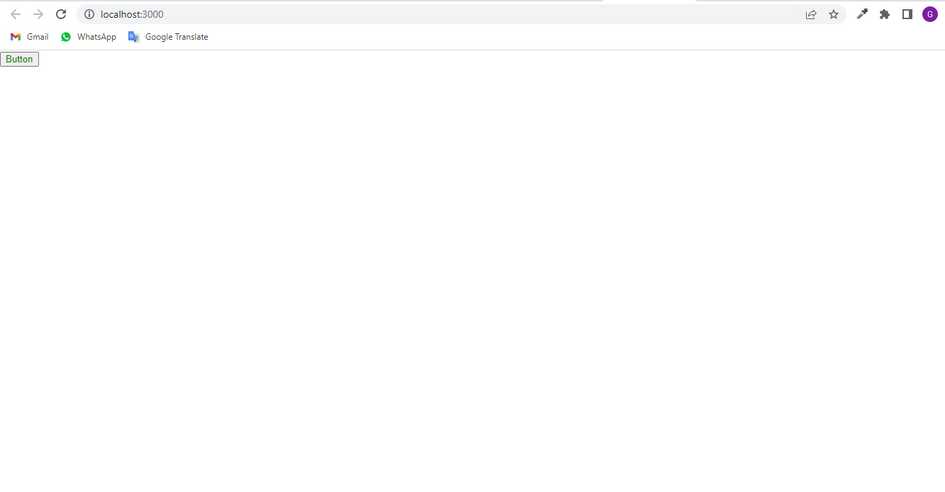This image depicts a minimalist web page interface. The body of the web page is completely blank, providing no additional content. At the top, in the browser’s tab section, there are several standard navigation icons: a left-facing arrow (back), a right-facing arrow (forward), a refresh button, and an address bar that contains an information ("i") icon and the address "localhost:3000." Toward the far right of the tab bar, there's a "send" button (which might be for a specific browser action) and a star icon typically used for bookmarking. 

Further to the right, there are four unidentified icons followed by a purple circle containing a white "G." Below this circle is the Gmail logo accompanied by the text "Gmail," followed by the WhatsApp logo with the text "WhatsApp," and then the Google Translate logo with the text "Google Translate." Below these icons, there is a thin gray horizontal line. At the bottom of the web page, there is a green button with the text "Button" inside it. Overall, the page appears to be a very basic layout, likely for testing or development purposes, given the address "localhost:3000."